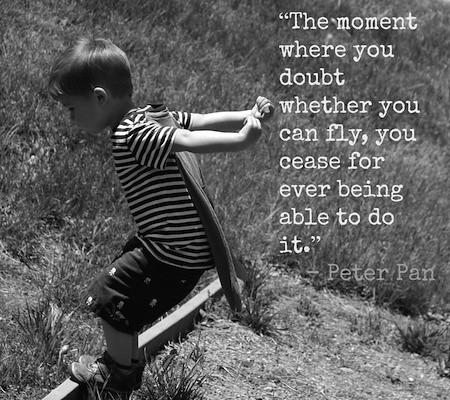In this evocative black-and-white photograph, a young boy, approximately three to five years old, is caught in mid-action, poised to leap off a small wooden 2x4 plank. He stands in a patchy grass field under the daytime sun, creating a nostalgic and timeless feel. The boy, dressed in a striped shirt, dark shorts, and small boots or tennis shoes, strikes a classic pose with his short, light hair and light skin. His arms are dramatically extended behind him as he pretends to fly, aided by a cape that flows from his shoulders—mirroring the whimsical spirit of Peter Pan. The side perspective of the photo adds a dynamic quality, emphasizing his intent to launch himself into the air. Overlaying the image, a poignant quote reads: "The moment where you doubt whether you can fly, you cease forever being able to do it. - Peter Pan," capturing the essence of childhood imagination and daring.